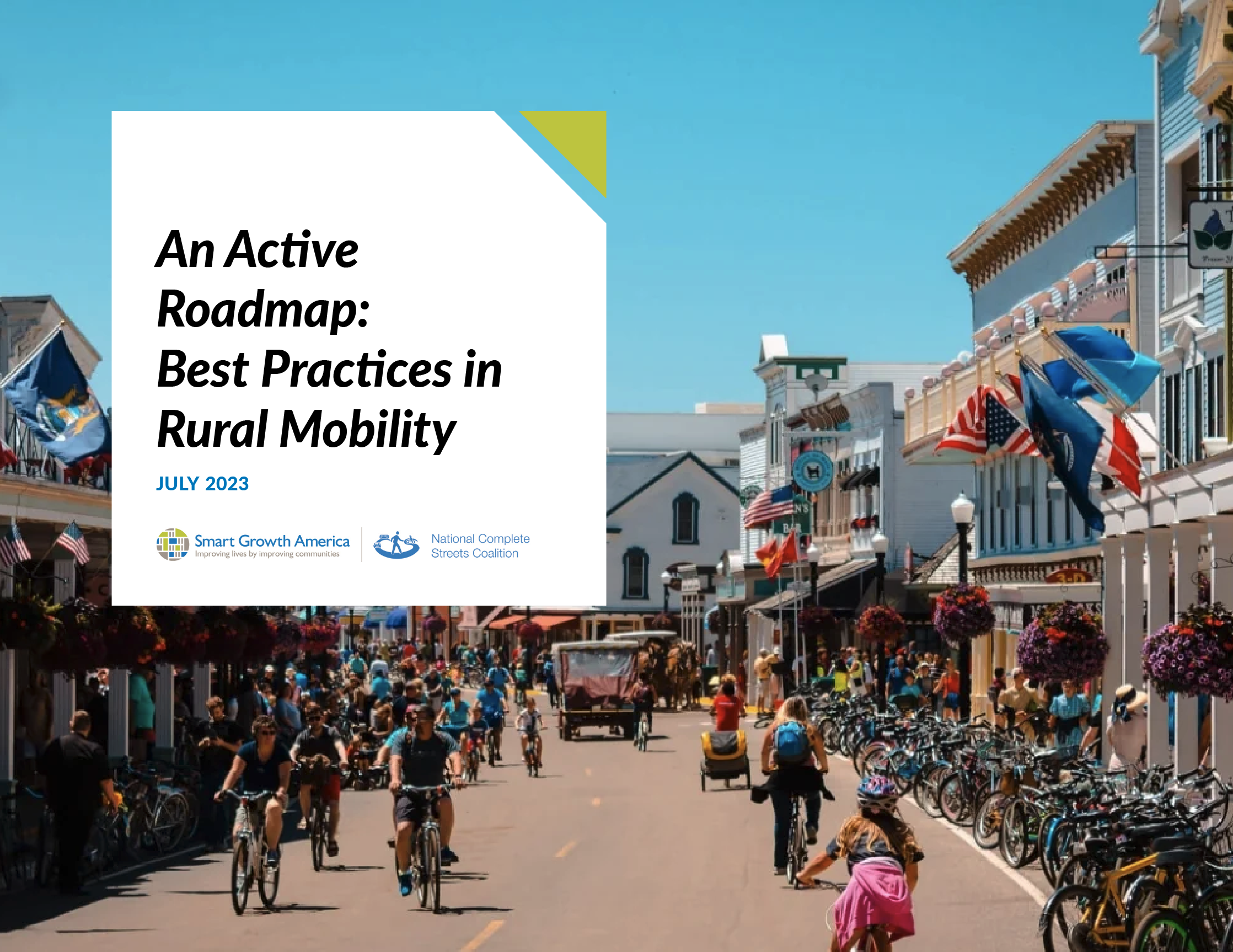The photograph captures a bustling small-town street scene during what appears to be a significant community event centered around bicycles. The street, a two-lane road flanked by multi-storied buildings, is teeming with activity. Bicycles dominate the scene, with many parked neatly along the sidewalks and numerous people of all ages and genders riding down the street. Pedestrians are scattered about, adding to the lively atmosphere. The buildings are adorned with various national flags, including American and Brazilian, suggesting a diverse and inclusive celebration.

In the upper left corner of the image, a large white square overlay displays text that reads: "An Active Road Map: Best Practices in Rural Mobility," dated July 2023 and attributed to Smart Growth America in collaboration with the National Complete Streets Coalition. The event seems designed to showcase rural mobility best practices, although there is a sense of critique from some onlookers who feel the initiative imposes external views on local lifestyles.